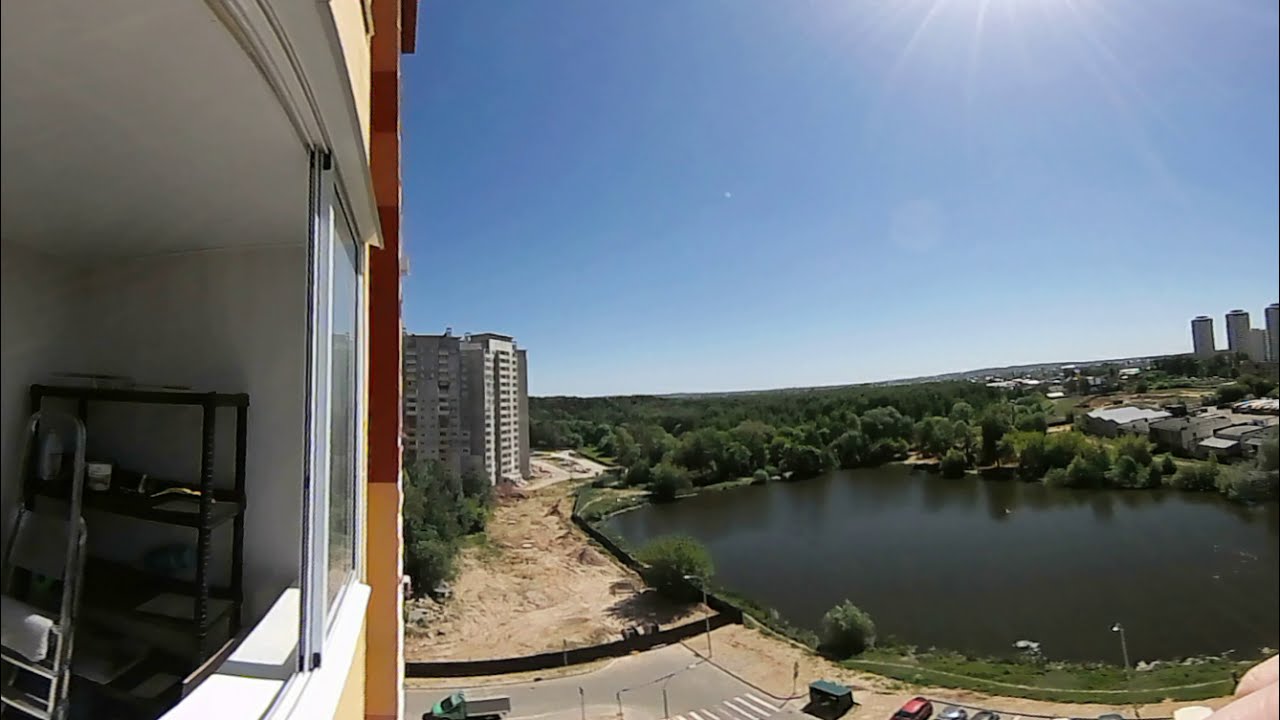This photograph, taken from an upper floor of a building, captures a slightly fisheye view of a cityscape centered around a circular, dark green pond or small lake shaded by reflections from surrounding trees. To the right of the pond, there are tall residential buildings, about three distinct multi-story structures, indicating a city environment. The foreground reveals a parking area with several parked cars under the bright, cloudless blue sky, with just the sun's rays peeking in from the top right corner, suggesting early evening light. To the left, the image shows an up-close view of a somewhat run-down building with open windows and a room containing a step ladder and storage shelves. Some sandy terrain, possibly a construction site, lies in front of a tall, grey concrete residential building, which contrasts with the dense forest stretching across the background center. The overall composition highlights the coexistence of urban architecture and natural elements within this city setting.